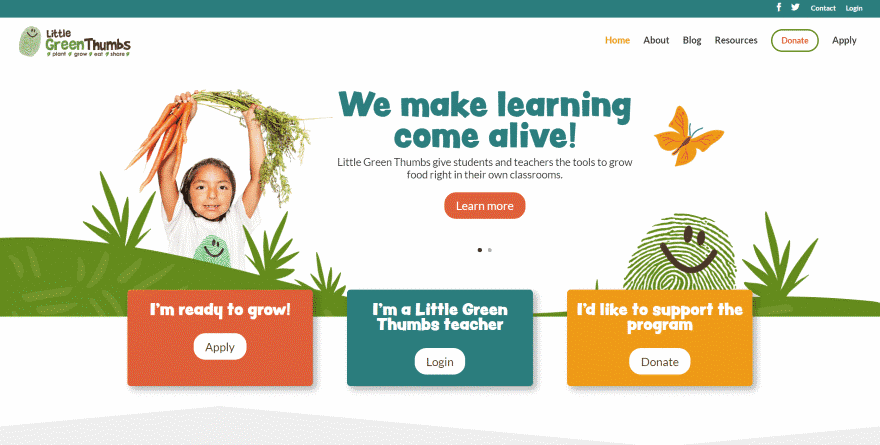The page features a clean white background, topped with a slender dark green banner. Below this banner is a graphic of a smiling green thumb. Adjacent to the thumb are the words "little green thumb," with "little" in brown, "green" in bold green, and "thumb" in bold brown letters. Beneath this, the text "plant, grow, eat, and share" is displayed.

On the right-hand side of the page, navigation tabs are present. The "Home" tab is highlighted in yellow, while the "About," "Blog," and "Resources" tabs are in black. There is a red-circled tab labeled "Donate" in red letters. The following tab, "Apply," is also in black letters.

At the center of the page is a captivating image of a child wearing a white t-shirt adorned with a small green thumb icon. The child, likely a Spanish boy with dark hair, proudly holds freshly harvested, long, and beautiful orange carrots. The child displays the carrots with the orange parts held high in his right hand and the green tops in his left hand.

Inside the picture, a green text overlay reads, "We make learning come alive. Little Green Thumbs gives students and teachers the tools to grow food right in their own classrooms."